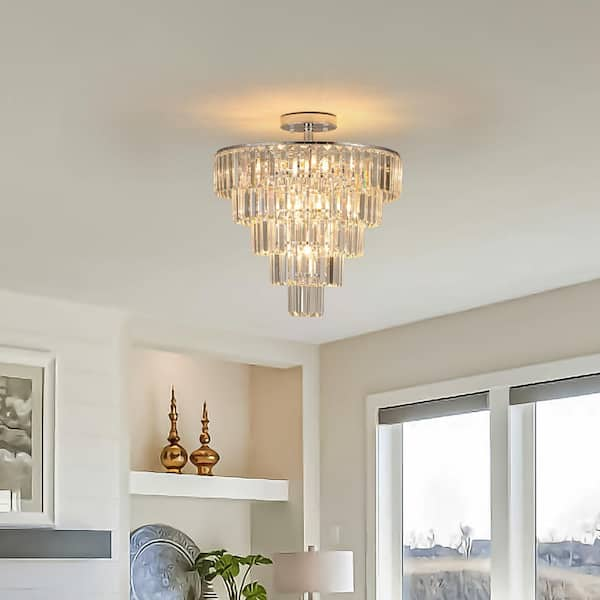The image captures an interior room with an upward perspective towards the ceiling's corner, providing a comprehensive view of the space. Dominating the scene is a crystal chandelier, emitting a warm yellowish-orange light. This chandelier, composed of several tiers, has a design that forms an inverted pyramid or an upside-down triangle, with five layers of concentric circles that diminish in size towards the center. The chandelier's crystals appear as strips or flat, wide pieces, and while giving a crystal-like appearance, they may likely be plastic.

The room itself is painted white, contributing to a bright and airy ambiance. On the right wall, there's a sliding glass door with a white frame, allowing a glimpse of the outdoors in daylight. On the left wall, built-in shelves house various decorations, including pointy pots, brass finials, a metallic plate, and part of a lamp and picture can be seen. These elements add character to the otherwise monochromatic space. The focal point remains the intricate chandelier, hanging from the ceiling and casting its light elegantly throughout the room.